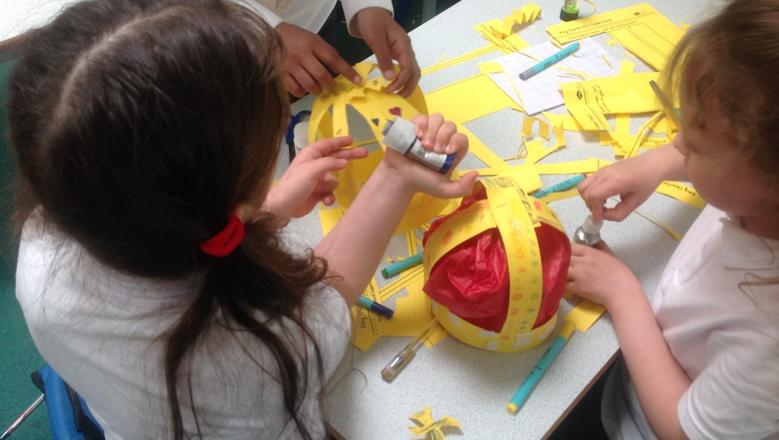The overhead color photograph captures a vibrant scene of children engaged in an art project, meticulously crafting crowns. The centerpiece is a nearly completed crown, featuring a red velvet-like base made from squishy tissue paper, intersected by a gold band and yellow construction paper, adorned with little fake gemstones. Scattered around are various colored markers and tubes of glitter glue, suggesting the intricate detailing that the children are adding to their creations.

In the left forefront of the image, a young girl with dark hair tied in pigtails by red bands dominates the frame. Dressed in a white shirt, she is engrossed in squeezing paint from a tube. Nearby, there are visible adult hands, likely those of an African American art teacher with long sleeves, assisting in the delicate process of gluing and arranging the elements of the crown.

On the right side of the table, another younger child is also seen enthusiastically participating, using glitter glue to decorate. The activity unfolds on a laminate tabletop, with the children of varying ages contributing to the shared creative endeavor.